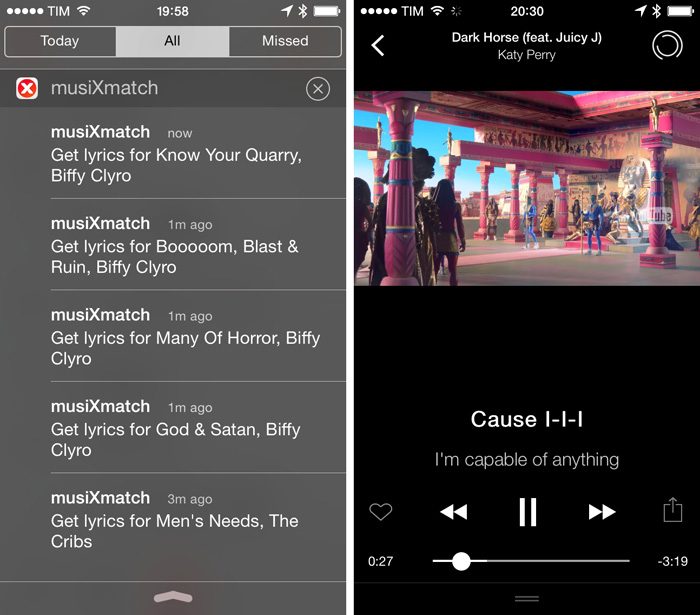This composite image consists of two screenshots from a mobile phone. 

**Left Screenshot:**
- **Background & Top Bar:** The background is gray. At the top, information about the phone is displayed in white font. 
  - **Top Left Corner:** Six large white circles displaying the carrier "Tim."
  - **Center:** The full Wi-Fi signal is prominently displayed, with the time shown as 19:58.
  - **Top Right Corner:** Indicators for location sharing and Bluetooth are turned on, and the battery is fully charged.

- **Notification Section:**
  - A gray web page features a rectangle at the top labeled "Today," "All," and "Missed," with "All" selected and highlighted in a lighter gray.
  - Below this, "Muse X Match" appears with a close button (X).
  - Multiple notifications from "Music Match" follow:
    - **Most Recent:** "Get Lyrics for Know Your Quarry" by Biffy Clyro, labeled "now."
    - **One Minute Ago:** "Get Lyrics for Boom, Blast and Ruin" by Biffy Clyro.
    - Other entries include "Get Lyrics for Many of Horror" and "Get Lyrics for God and Satan," both by Biffy Clyro.

**Right Screenshot:**
- **Web Player Interface:**
  - A song is currently playing, identified as "Dark Horse" featuring Juicy J by Katy Perry.

This detailed description provides a clear understanding of the content and layout of each screenshot.